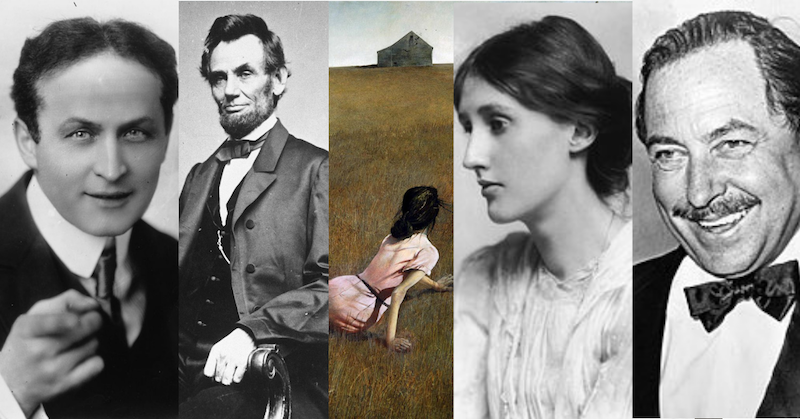The image is a composite of five vertically spliced panels featuring varied and striking figures from different times and contexts. On the far left is a black-and-white photograph of a man in his 30s, likely Harry Houdini, dressed in a suit and tie, pointing towards the camera with a determined expression. Next to him is another black-and-white photograph of Abraham Lincoln, dressed in a suit with his traditional beard, looking straight at the camera with his arm resting on a wooden banister. The central panel features a painting of a woman in a pink dress with medium-length brown hair, sitting sideways in a field of brownish prairie grass and gazing towards an old homestead house on the horizon. To the right of the painting is a black-and-white profile shot of a woman, possibly from the late 1800s or early 1900s, in a white dress, her dark hair pulled back in a bun, looking solemnly to the left. The final image on the far right is a black-and-white photograph of a man in his late 40s to early 50s, wearing a tuxedo with a bow tie, a short groomed mustache, and slicked-back hair. He has a warm, joyous smile, seemingly recognizing him as an actor from the early 20th century. Each section presents a unique slice of history and art, capturing distinct personalities and moments.